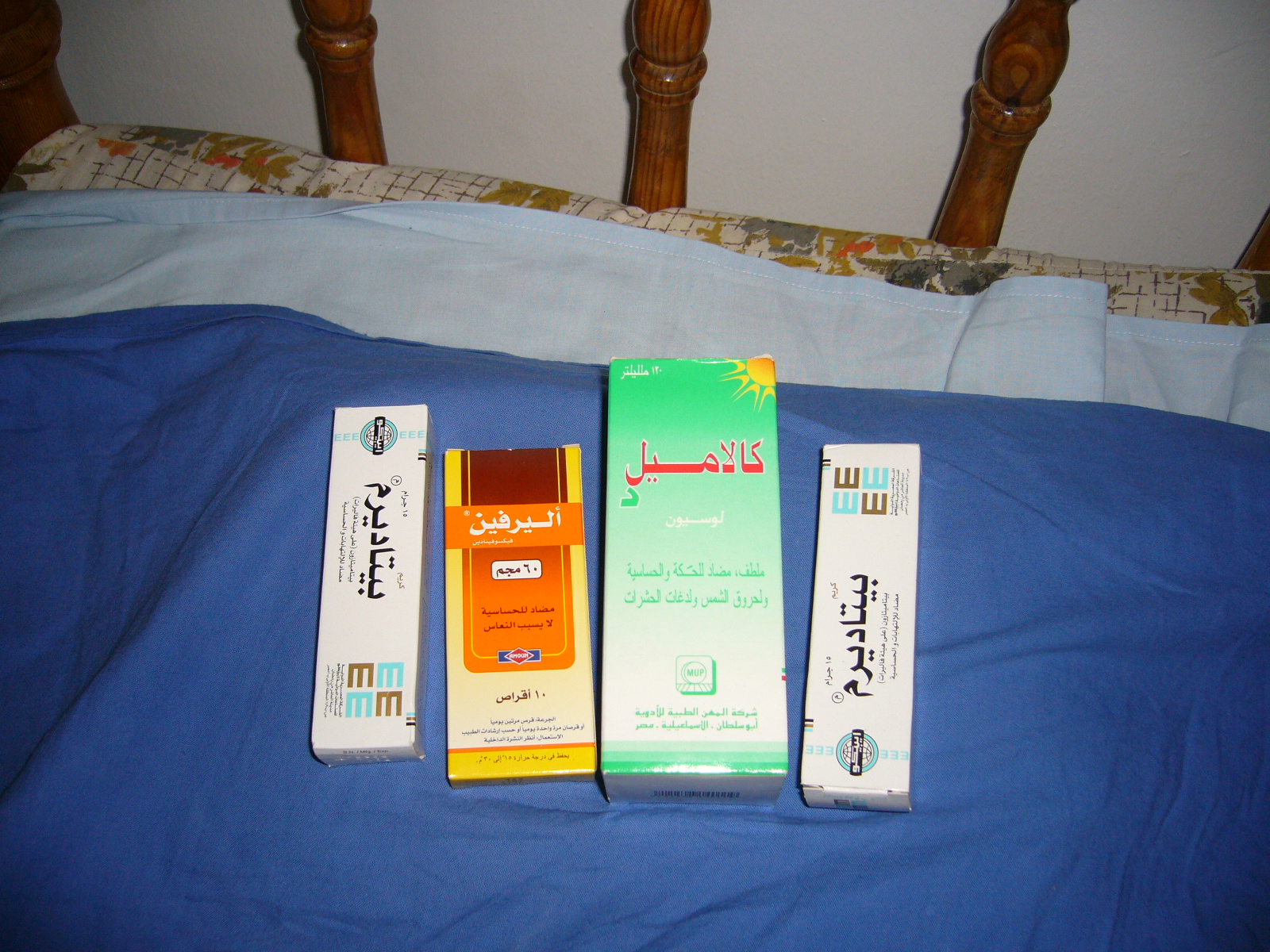The image depicts four rectangular boxes of various shapes, sizes, and colors, presumably containing medication, placed vertically on a blue bedsheet with a white comforter. In the backdrop, there are beige and gold floral-themed pillows or sheets, wooden bed railings with five vertical spindles, and a white wall.

1. The box on the far left is tall, rectangular, and white. It has several elements, including a brown and blue "M" logo, black script that appears to be in an oriental or Arabic language, and a blue circle with black writing. 
2. The second box is slightly shorter and predominantly yellow with orange and burgundy labels. It features white writing at the top, with more writing at the bottom that appears to be indecipherable.
3. The third box is the largest, about 20% bigger than the second. It has a green background with a yellow sun in the top right corner, red elements, and green writing that might be from a different language, possibly European.
4. The fourth box resembles the first but with inverted design elements, including the brown and blue "M" logo and black script.

Details of the bed setup and decoration, as well as the intricate box designs, suggest a meticulous arrangement, alluding to their unknown but likely medicinal purpose.